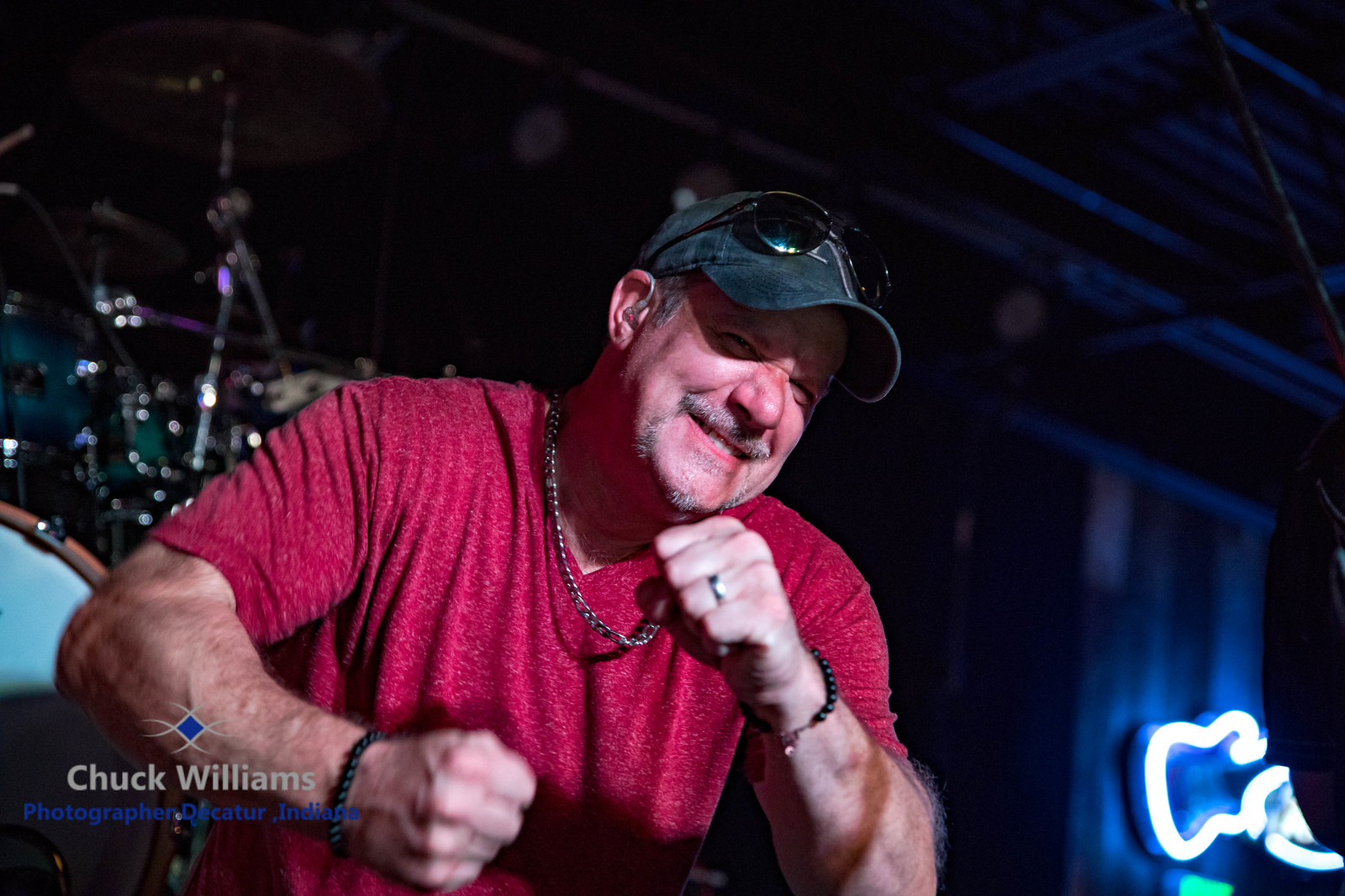A detailed photo captures a man standing on a dark stage, with a drum set visible on the left background and a neon LED sign of a guitar illuminating the bottom right corner. The man, who has brownish-gray hair and is white, is dressed in a short-sleeved red heather v-neck t-shirt. He wears a gold wedding ring, black bead bracelets on both wrists, and a silver chain necklace. His black ball cap, which has sunglasses resting on top, contrasts with his goatee and mustache. His fists are clenched, with one fist positioned near his chest and the other near his chin, while he smiles towards the camera. The photo includes a white and blue watermark in the bottom left corner, indicating the photographer's name, Chuck Williams, with the text "Photographer, Decatur, Indiana," and a diamond logo.